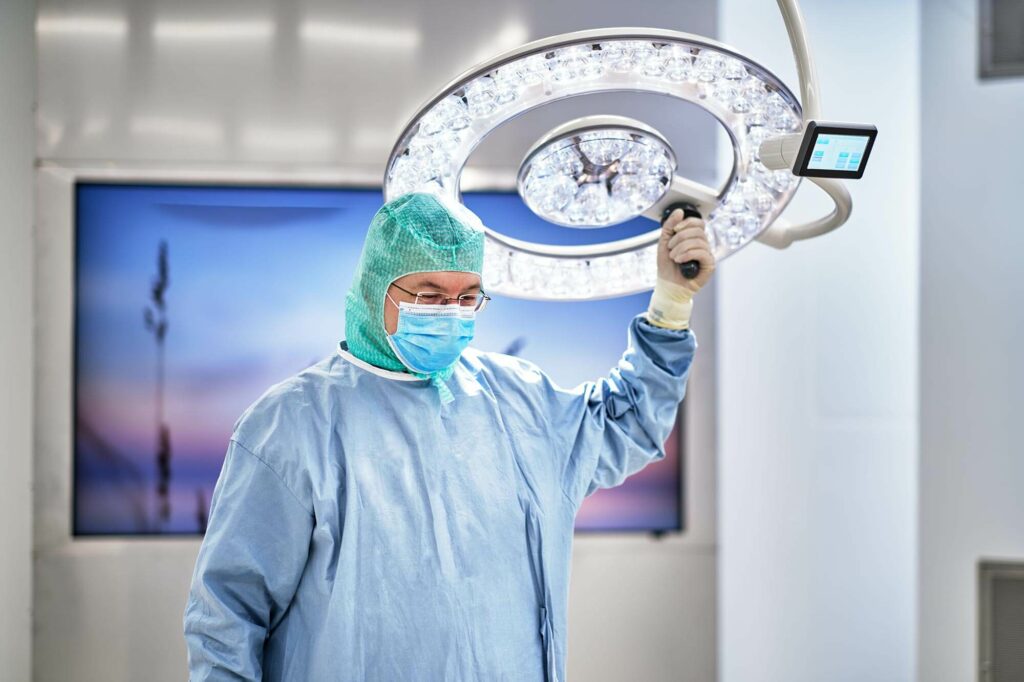In this brightly lit and possibly airbrushed photographic image, a man—presumably a surgeon—is standing in a pristine, white surgical suite. Clad in full personal protective equipment, he wears a blue surgical robe and a greenish-blue hood that covers his head and neck, leaving only his face exposed. His face is protected by a blue and white surgical mask, and he sports glasses. With his left hand, he is adjusting a large, circular overhead light, engineered with multiple bulbs encircling the outer part and a central cluster of lights. The light, mounted on a swivel arm, features a handle for easy maneuvering, ensuring optimal illumination of the surgical area. Attached to the light is a camera, perhaps for medical students to observe the procedure. The white walls of the room are adorned with additional lighting equipment, and behind the surgeon, there is a blurry yet sizeable flat-screen monitor. This detailed setup suggests a highly sterile and professional environment, essential for intricate medical procedures.